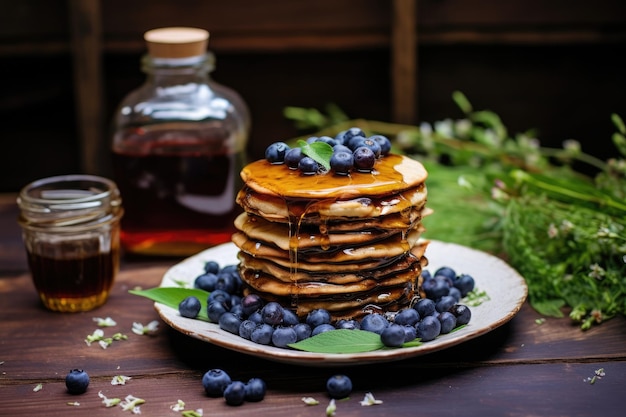This close-up food shot captures a tall stack of blueberry-topped pancakes, elegantly plated on a white dish with gold edging, set atop a rustic dark wood table. Syrup generously drips down the sides of the pancakes, enhancing their rich, golden-brown texture. The plate features a decorative array of fresh blueberries encircling the pancakes, interspersed with sprigs of mint. Additional blueberries are artfully scattered around the plate and on the table, adding a touch of vibrant color. In the blurred background to the left, a glass jar brimming with syrup is visible, along with a decanter sealed with a cork lid, both containing rich, amber-colored syrup. The overall presentation is further accentuated by the delicate placement of mint sprigs among the blueberries, making for a visually appealing and mouth-watering display.